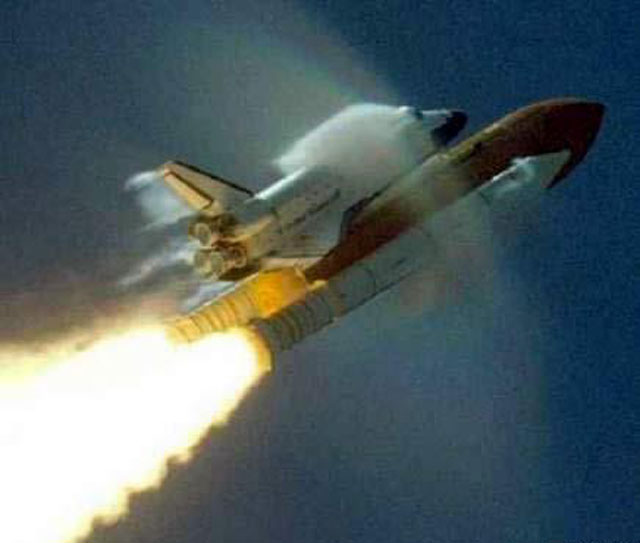A vintage, square photograph captures the dramatic moment of a space shuttle launch, though the image is somewhat blurry. Dominating the center of the photograph, the black and white space shuttle is attached to two white booster rockets and a central orange fuel tank. The photograph shows the shuttle launching diagonally from the bottom left corner towards the top right, against a backdrop of a dark blue sky. A misty, gray rainbow-like halo surrounds the shuttle as it pierces through the atmosphere. The boosters, each crowned with conical tips, emit vivid orange flames from their cylindrical thrusters. The shuttle features a conical nose and a distinct cockpit area, evidenced by a visible windscreen for the pilot. The rear exhibits a sizable fin and four unlit rockets, adding to the intricate details of this awe-inspiring launch.